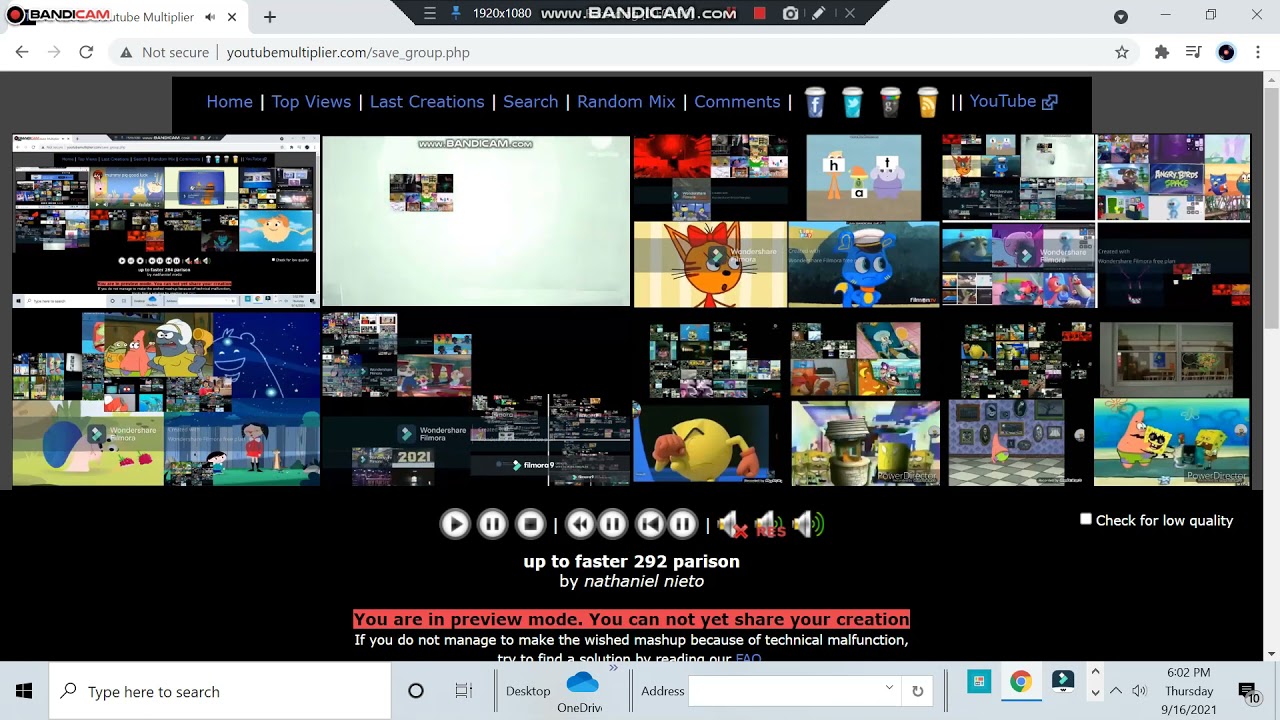**Detailed Caption:**

This screenshot captures a user’s Chrome browser open to a website called "youtube-multiplier.com." The main feature of this site is the ability to pair and play multiple YouTube videos simultaneously, visible by the assortment of video thumbnails and playback controls on the page. An overlay at the top of the browser window prominently displays "bandicam.com," indicating the use of Bandicam screen recording software. Additionally, the browser is shown with an unusually tall taskbar at the bottom of the screen, cluttering the view. The taskbar displays various open applications and system icons, adding to the overall busy and somewhat chaotic appearance of the screenshot.